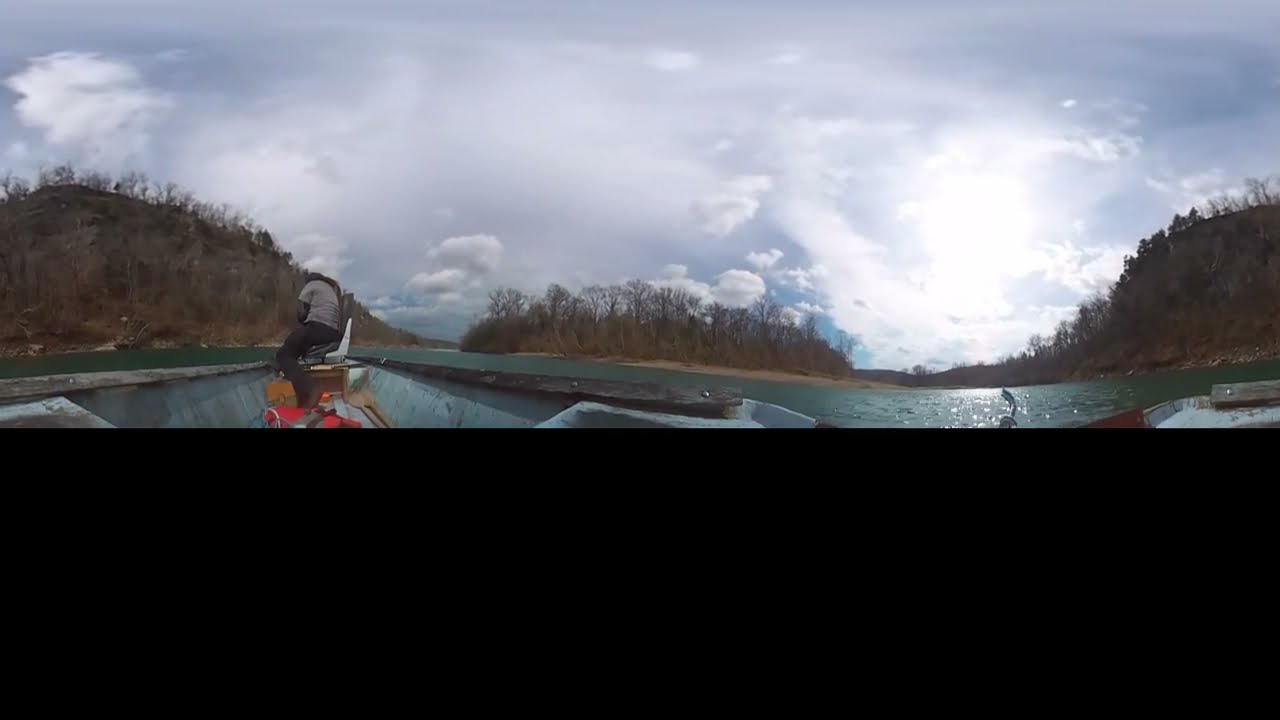This is a detailed, panoramic image showcasing a serene river or lake landscape during a cloudy fall or winter day. A man, wearing a gray shirt or jacket and black pants, is seated on a white chair at the bow of a small metal fishing boat, approximately 15 to 20 feet long. The boat contains various fishing equipment, including oars, an orange life preserver, and other essentials. The hull features a wood railing with silver rivets around it. The man's face is obscured as he looks over the edge of the boat, seemingly engrossed in fishing. Surrounding the calm, blue water are numerous hills and bare trees, indicating the season. The shorelines and inlets suggest the waterway forks or provides multiple navigation routes. The image's 360-degree distortion is evident from the curved lines throughout the scene. The photograph is framed with a thin black border at the top and a wider black border at the bottom, contributing to its panoramic feel.